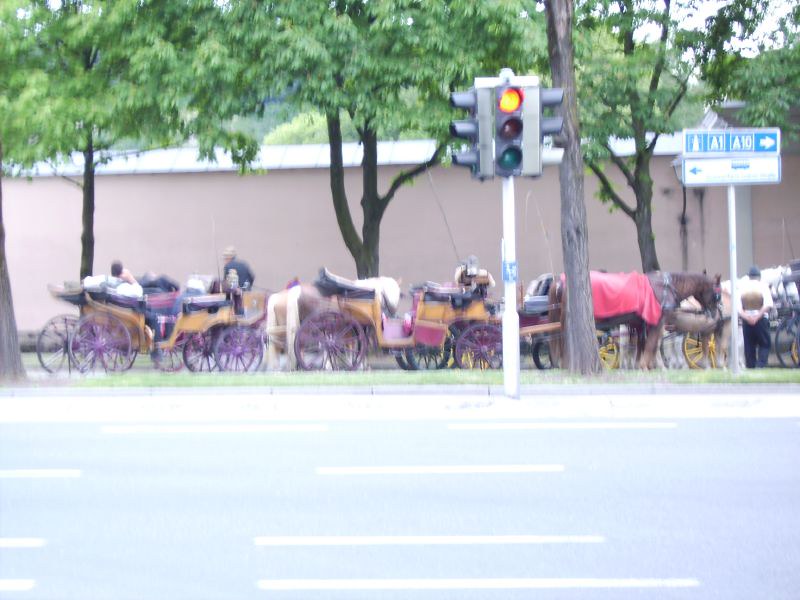This photograph captures a modern urban street scene featuring a collection of old-fashioned horse-drawn carriages amidst a backdrop of lush trees and an expansive beige building. In the foreground, a three-lane road extends up to roughly 40% of the image, devoid of traffic. Prominently positioned in the middle of the scene is a traffic light, which shows a red signal from the viewers' perspective. Flanking this traffic light to the right stands a blue and white street sign, adjacent to a sizeable tree with dense foliage. In the background, four carriages are aligned along the pavement. These carriages mostly appear to have brown-colored bodies, with one notably adorned with a blue top and purple wheels. One horse, draped in a red blanket, is visible, while another hides partially behind it. The scene also includes a few indistinct figures, hinting at onlookers or potential passengers. The grandeur of the beige building stretches across the width of the scene, complemented by additional tree canopies peeking over its rooftop. The overall composition melds the charm of traditional carriages with modern urban elements, creating a captivating contrast.